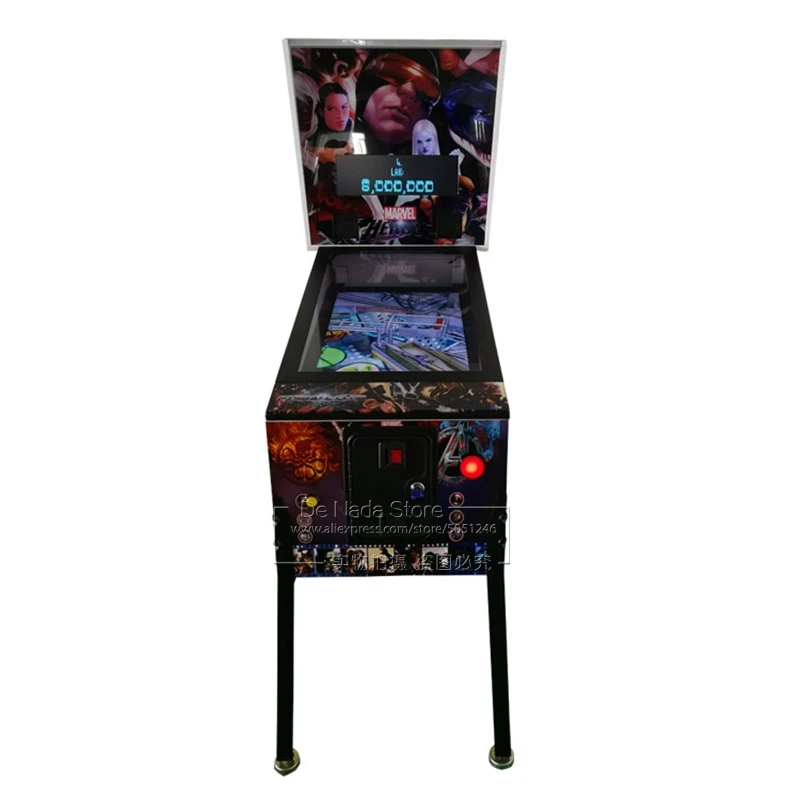The photograph captures a detailed image of an arcade machine, which has a decidedly retro, pinball-like appearance. The main body of the machine is cuboidal and metallic, with intricately decorated outer surfaces featuring colorful drawings and paintings. Notably, a prominent poster is affixed to the front of the machine, showcasing faces of cartoon or superhero characters, with "MARVEL" written below a blue numerical score—stated alternately as 6,000,000 or 8,000,000. The machine includes a large vertical screen at the top displaying the score in blue lights, while the lower section features a semi-transparent blue and red screen on a flatter panel, along with various lit buttons in red, blue, and yellow. The legs of the machine are straight and black. Dominating the middle of the image is a semi-transparent watermark reading "BI LADA STORE www.aliexpress.com" in addition to other characters. The background is a plain white, providing clear visibility of the machine's features.